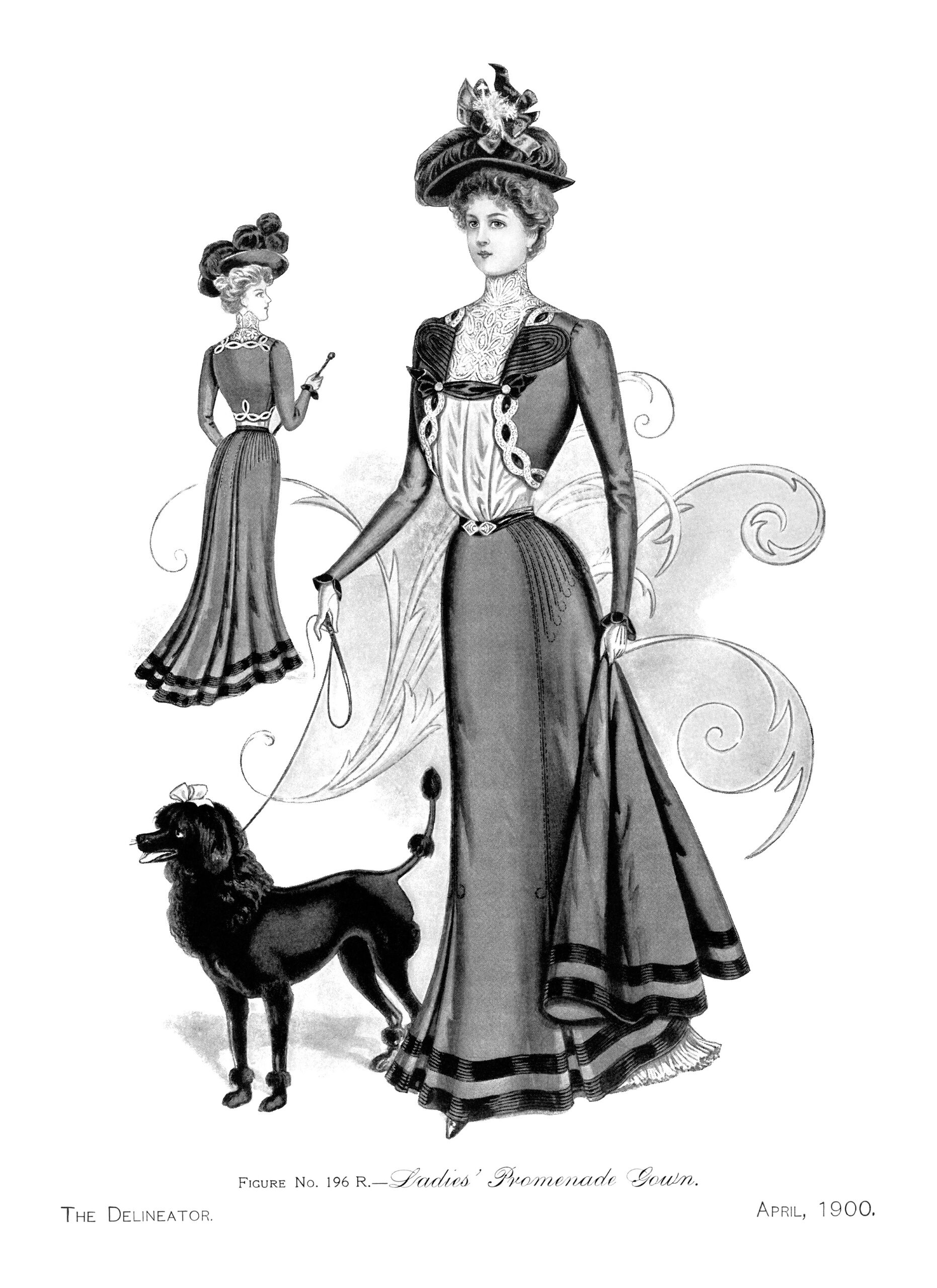This black and white hand-drawn illustration from April 1900, as noted by the text "Figure Number 196" at the bottom, features a detailed portrayal of a woman in Victorian-era attire. At the forefront, a tall woman with her hair neatly pulled up is adorned in an elegant long-sleeve dress. The dress boasts intricate details such as black frilly cuffs, a white, frilly design down the front of her chest, and two black borders adorning the hem. She is accessorized with a large, ornate hat decorated with elements resembling flowers, feathers, and possibly a small bird. In her right hand, she holds a leash attached to a black poodle, characterized by puffs on its tail and a bow in its hair. To the left, a smaller rear view of the same woman is depicted, providing a comprehensive view of her elaborate outfit, including her hat and the back design of her dress. The background features a curly, swirly design in shades of gray, complementing the overall aesthetic of the image and emphasizing its historical and artistic attributes.